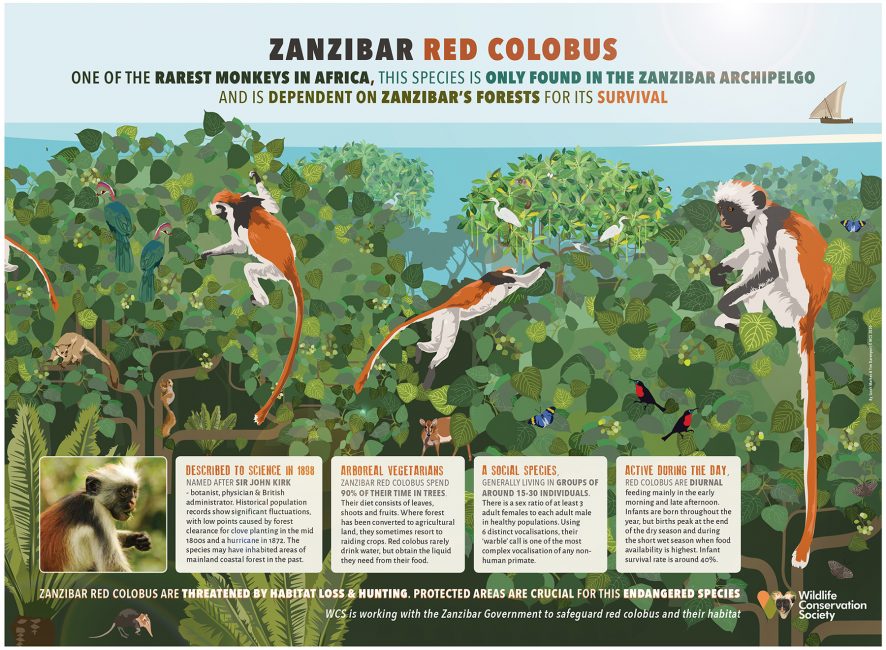This informational poster highlights the endangered Zanzibar red colobus monkey, one of the rarest monkeys in Africa found only in the Zanzibar archipelago and dependent on its forests for survival. Dominating the image is a detailed watercolor illustration featuring three Zanzibar red colobus monkeys with distinctive orange backs, black faces, white trimmings around their faces and ears, and long tails with white undersides and brown-orange tops. These monkeys are depicted leaping through lush, leafy trees amidst abundant foliage. The background includes an array of wildlife, such as deer, squirrels, red birds, and storks. In the distant background, there's an ocean with a sailboat gliding across it. Below the illustration, there is a photograph of a real Zanzibar red colobus, adding a touch of realism. Adjacent to this photo are four informational boxes with headings on scientific classification, dietary habits, social behavior, and daily activities of the monkeys. Additional text emphasizes the threats of habitat loss and hunting faced by the Zanzibar red colobus, calling attention to the crucial protected areas. The Wildlife Conservation Society's logo, consisting of two hearts, is in the bottom right corner, underscoring their efforts in working with the Zanzibar government to safeguard these endangered primates and their habitats.